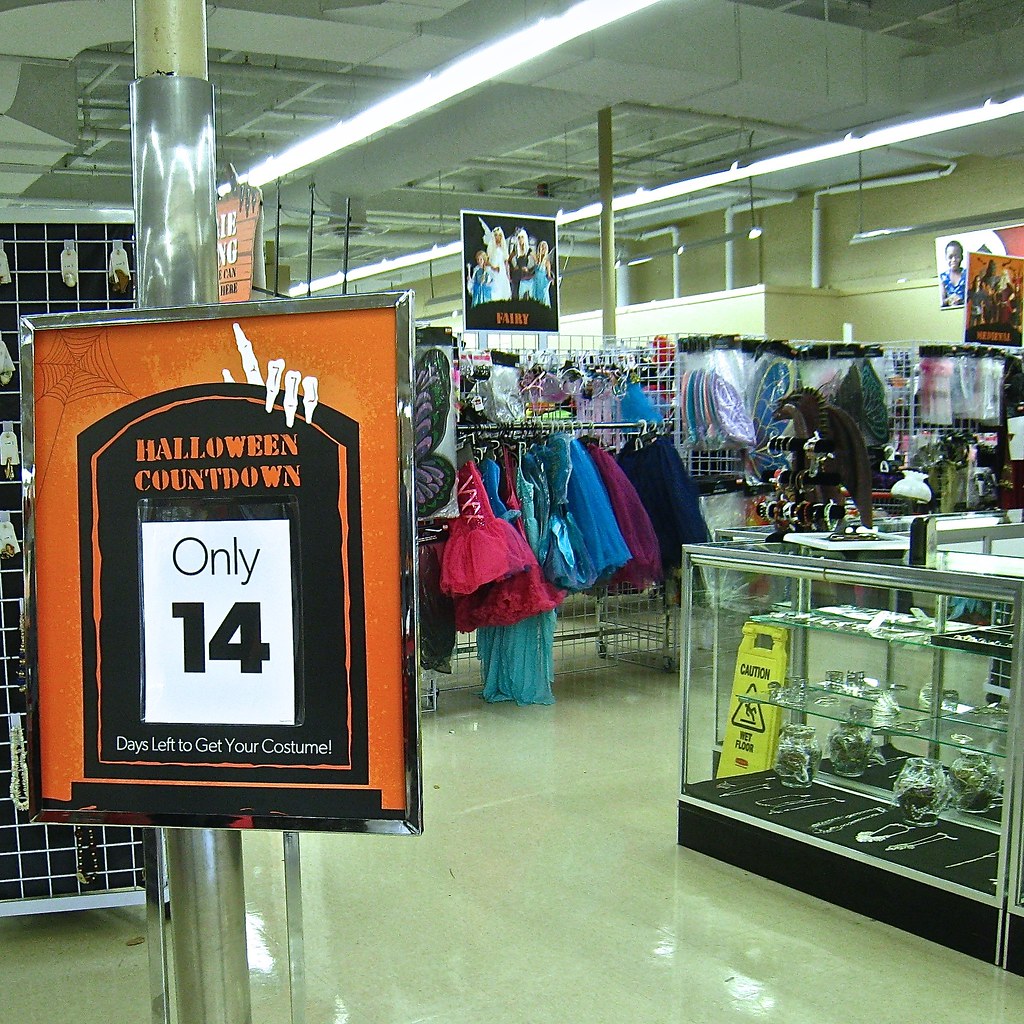This photograph captures an angled view of a large and diverse costume store. Dominating the left side of the image is a prominent silver-framed sign with an orange background, featuring a black headstone graphic that reads "Halloween Countdown" in large orange letters. A smaller piece of paper within a plastic pocket indicates "only 14" days left to get your costume, with the message in small white letters at the bottom. To the right, a glass display case is filled with an assortment of costume accessories like necklaces and tiaras. Moving towards the background, a sign hangs from the ceiling depicting children dressed as fairies, with the word "Fairy" prominently displayed in orange against a black background. Below the sign, racks are filled with fairy-themed costumes, including colorful pink, blue, and purple dresses and sets of butterfly wings. The store exudes a festive, organized atmosphere, dedicated to celebrating Halloween with a rich variety of costume options.